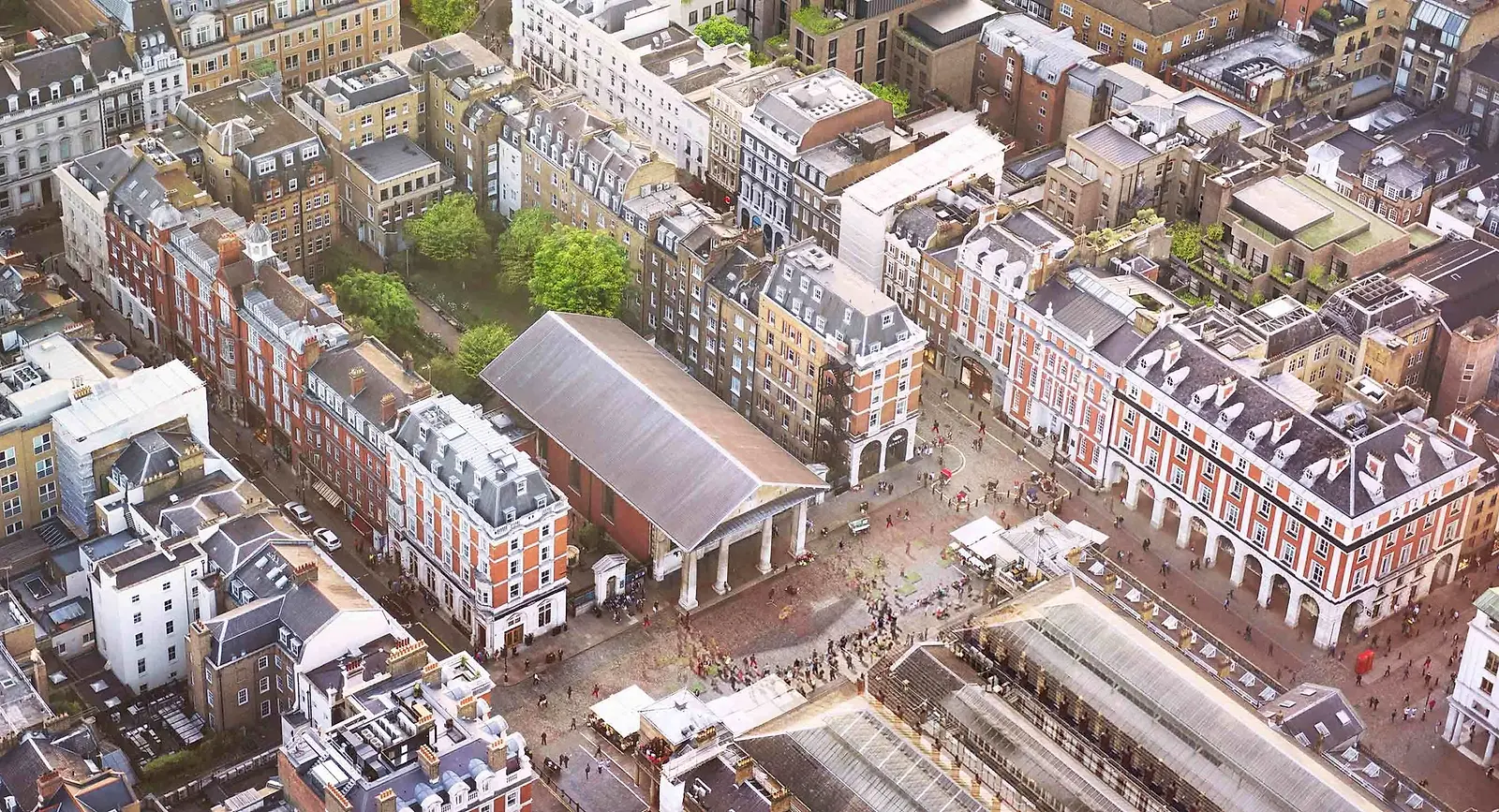This aerial photograph captures a vibrant cityscape reminiscent of London's architecture, focusing on an area that could easily be mistaken for a college campus or a lively city square. Central to the image is a long, rectangular, red-brick building featuring a distinctive four-arched portico, suggesting it might serve as a city hall or a significant campus building. This building is surrounded by a mix of multi-story apartment and residential buildings, primarily in red and brown brick, arranged in a horseshoe shape. The area within this horseshoe includes lush, lime-green trees indicative of early spring and possibly a small park or courtyard, with benches and open spaces where people gather and walk.

Further details reveal additional infrastructure: a train station or depot with long roofs located towards the lower section of the image, and a semi-circle of people in front of the portico, hinting at a performance or gathering. The upper left and right corners of the photograph show clusters of similar multi-story buildings, some with flat roofs and rooftop air conditioners, adding to the diverse cityscape. The absence of cars and abundance of pedestrians reinforce the area's vibrant, interactive atmosphere, making it a bustling hub filled with architectural charm and communal spaces.